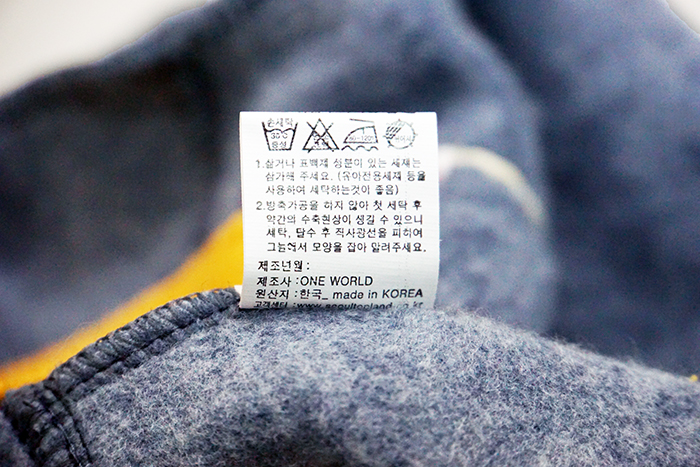This photograph features an extreme close-up of a clothing label, partially legible, attached to a garment that appears blue with a fluffy nap, possibly made of cotton or wool. The prominent white tag is primarily inscribed in Korean, which includes washing instructions illustrated by universal laundry symbols. Interspersed within the Korean text, some English words are visible: "One World" and "Made in Korea," followed by a website link. While the detailed content of the label remains obscured to those who cannot read Korean, the visible elements suggest standard garment care instructions. The rest of the garment remains out of focus, leaving its full appearance indistinct.